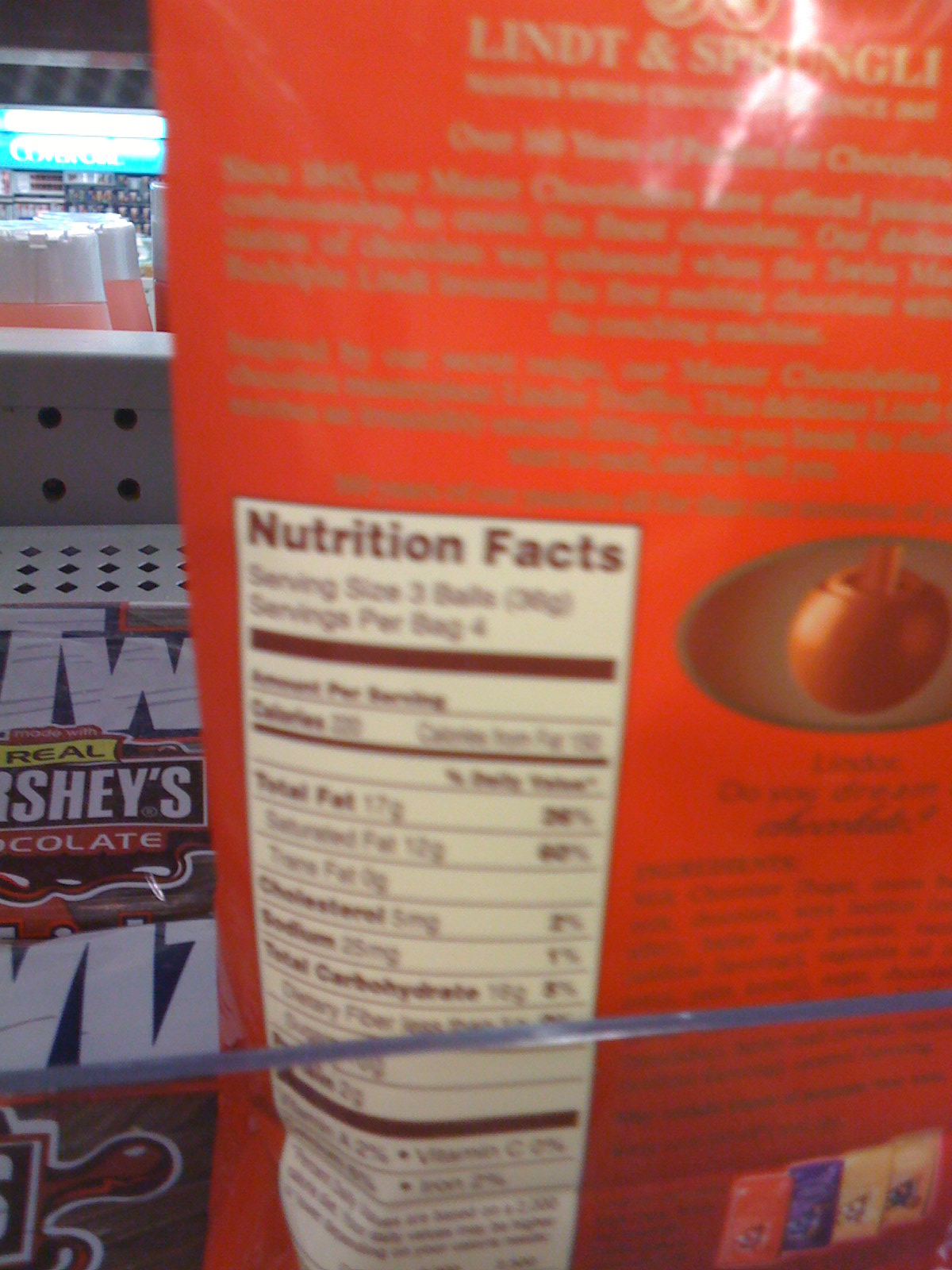This close-up photograph captures the back of a food product's packaging, though it is somewhat out of focus, making it challenging to identify the exact item. The packaging displays an image of chocolate being poured into small candy shapes. From the visibly discernible letters, it appears to be of the Lindt brand, as suggested by the partially visible "L," "I," "N," "D," and "O," "N" letters. Below the main image, the package illustrates various other packaging colors including red, blue, gold, and brown, showcasing the assortment of treats available from this brand. Although the photograph is blurry, the left side of the packaging hints at the presence of nutritional information with the words "Nutrition Facts" perceptible, indicating serving sizes and other details. In the background, just before the left edge of the photo cuts off, part of the store's interior can be seen, including shelving where the product is displayed.